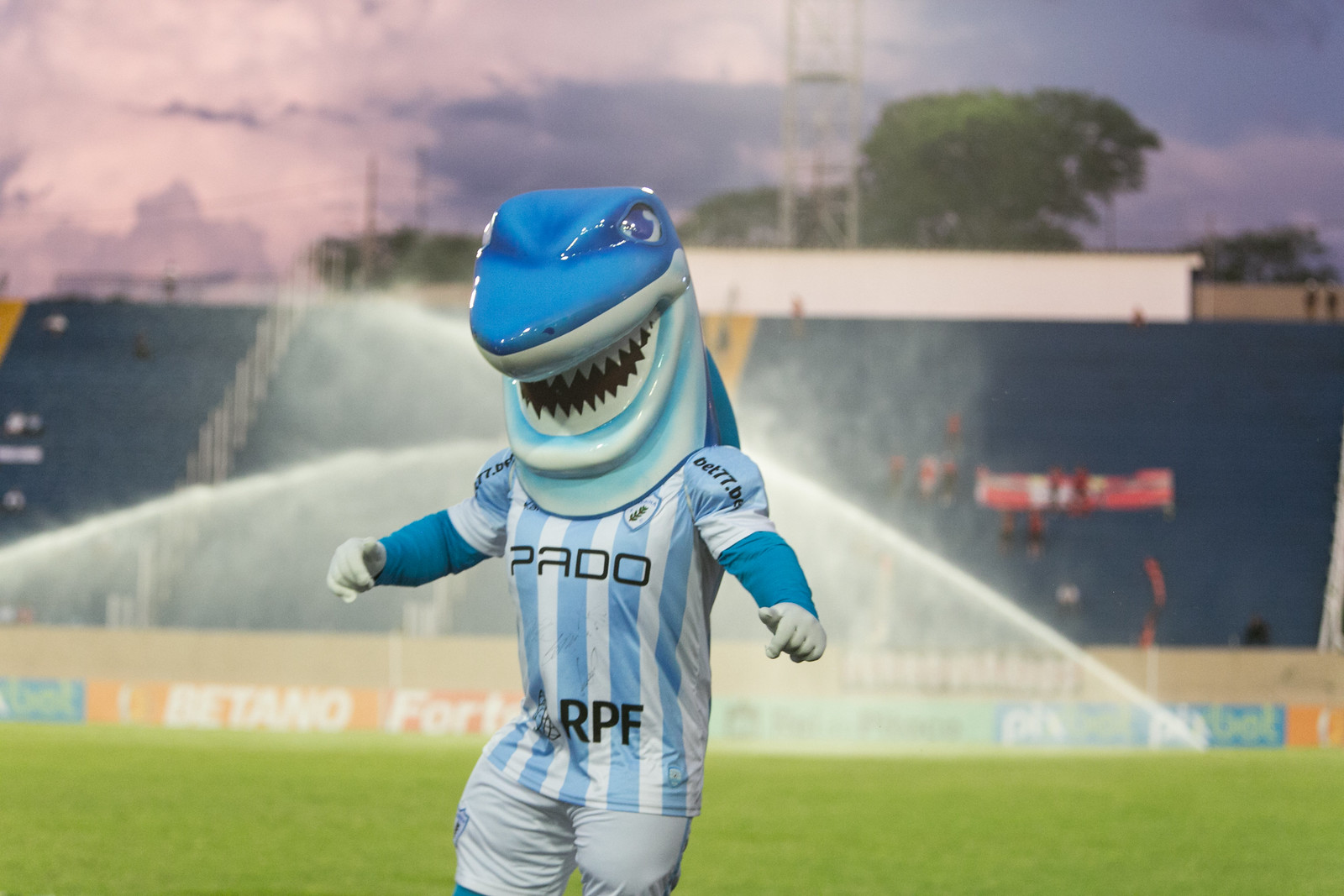In the foreground of the image, the sports team's mascot stands out vividly, a dynamic figure dressed in a distinctive white and blue vertically striped jersey adorned with large shoulder pads. The mascot is also outfitted in blue sleeves and white gloves, paired with gray shorts that have visible padding underneath. The centerpiece of the costume is an elaborate fiberglass shark head mask; this blue shark head is cartoonish yet fearsome, featuring big eyes, an open mouth bristling with sharp white teeth, and a fin that extends from the top and curves down the back, resting on the wearer's shoulders.

The background reveals a lush green soccer field drenched by multiple active sprinklers, shooting arcs of water across the scene. To one side of the field are stands with sections of white, blue, and yellow seating, interspersed with silver railings and overgrown trees. The broad, fluffy clouds in the sky range from subtle gray to a mix of blue and purple hues. Additional details include a wall behind the bleachers that is noticeably white, along with an audience holding red and white signs. Among the crowd, some viewers are dressed in red. Amidst these vivid background elements, the mascot's jersey is marked with "Pato" and "RPF" in black letters, completing the striking and immersive scene.